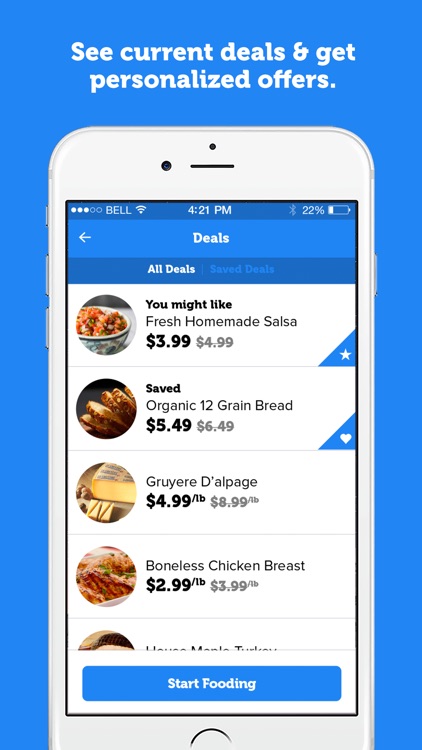Image Caption: 

The image features a blue background adorned with white text at the top. Central to the image is a depiction of a white smartphone displaying various pieces of information. At the top, the text reads "See Current Deals and Get Personalized Offers". 

The visible portion of the smartphone screen shows details typical of a mobile interface: the carrier is noted as "Bell", current time is 4:21 PM, and the battery level is at 22%. The device indicates Wi-Fi connectivity and Bluetooth activation. directly underneath the status bar, a left-pointing arrow is labeled "Deals", hinting at navigation options.

The section titled "Deals" highlights two categories: "All Deals" and "Saved Deals". "All Deals" is emphasized with white text on a blue background, whereas "Saved Deals" is blue text on the same blue background. Further down, a list of available deals is presented, though the fifth item is partially cut off. 

The deals are as follows:
1. **Homemade Salsa** - Priced at $3.99, previously $4.99 (struck through). This item features a blue icon with a white star.
2. **Organic 12 Grain Bread** - Priced at $5.49, previously $6.49 (struck through). This deal includes a blue icon with a white heart.
3. **Whole Deli-Ham Page** - $4.99 per pound, originally $8.99 per pound (struck through). A blue icon with a white heart is attached to this offer.
4. **Boneless Chicken Breast** - Priced at $2.99 per pound, reduced from $3.99 per pound (struck through). A similar blue heart icon is present.

The smartphone’s interface design and information presented suggest a promotional section within a mobile application dedicated to grocery deals or similar retail offers.